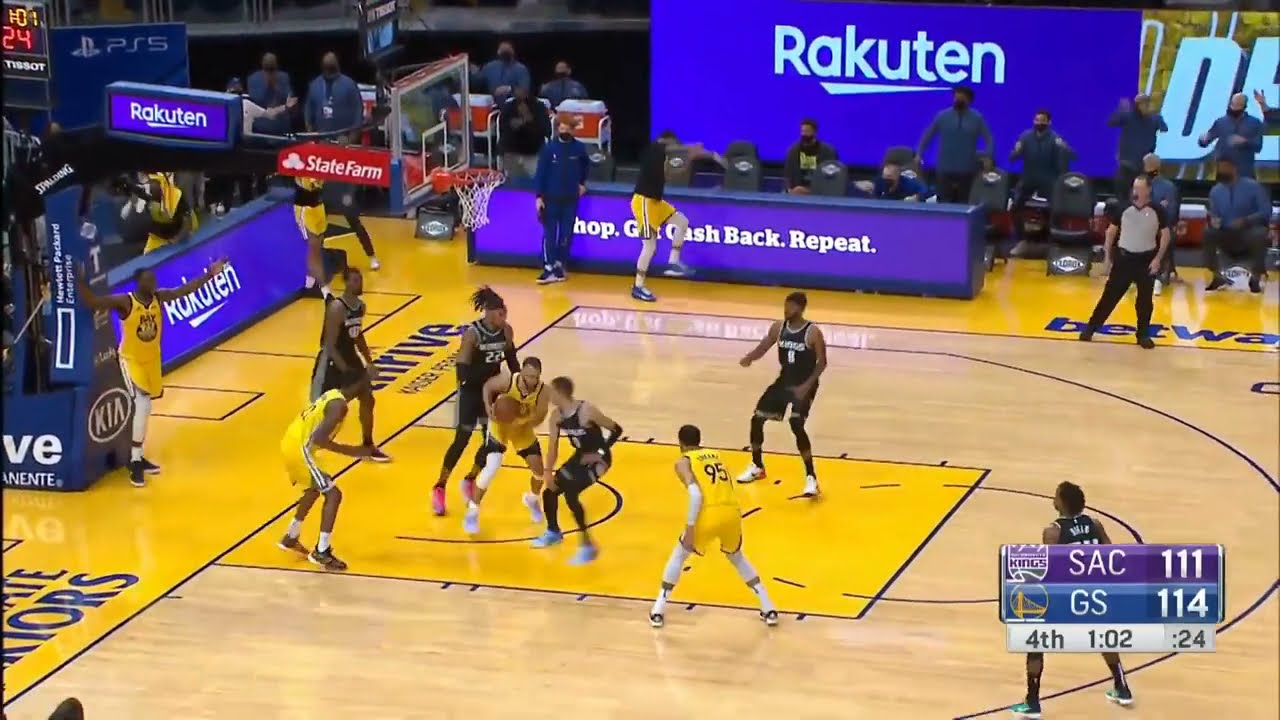A detailed image captures the intense moments of a live basketball game between the Sacramento Kings and the Golden State Warriors, as indicated by the TV scoreboard graphic. The action occurs in the fourth quarter with 1:02 remaining and the shot clock showing 24 seconds. The Golden State Warriors lead with a score of 114 against the Kings' 111. Half of a light brown wooden court with a bright yellow painted area under the hoop occupies the frame. The hoop, adorned with advertisements for State Farm, Rakuten, and PlayStation 5, emerges from the top left corner.

Players from both teams, distinguishable by their uniforms—yellow and white for the Warriors, black and white for the Kings—are actively engaged in play. One Warriors player is holding the ball near the hoop, closely guarded by two Kings players. The crowd in the background, visible alongside the court and in the stands, cheers on enthusiastically. The arena is decked with various advertisements, particularly the bright purple Rakuten ads with white lettering stating "Shop, get cash back, repeat," prominently displayed on the barricades and walls. The presence of referees, the vibrant atmosphere, and detailed court elements paint a vivid picture of this high-stakes NBA game.